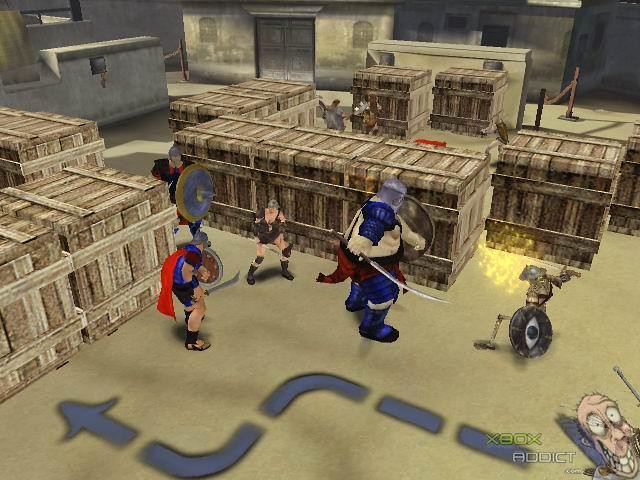The image showcases an Xbox game, possibly titled "Addict," as indicated by lettering on the screen's bottom right. The game's visual setting appears to be medieval, featuring a group of armor-clad men wielding large round shields and hefty swords. The scene takes place inside a dimly lit warehouse filled with wooden crates, some of which are marked with directional arrows, suggesting they could be interactable objects or hiding points for treasures. The backdrop of the warehouse comprises sturdy stone walls and several doorways, further emphasizing the historical ambiance. The precise objective of the game remains unclear, but the imagery hints at exploration or treasure hunting in a bygone era.